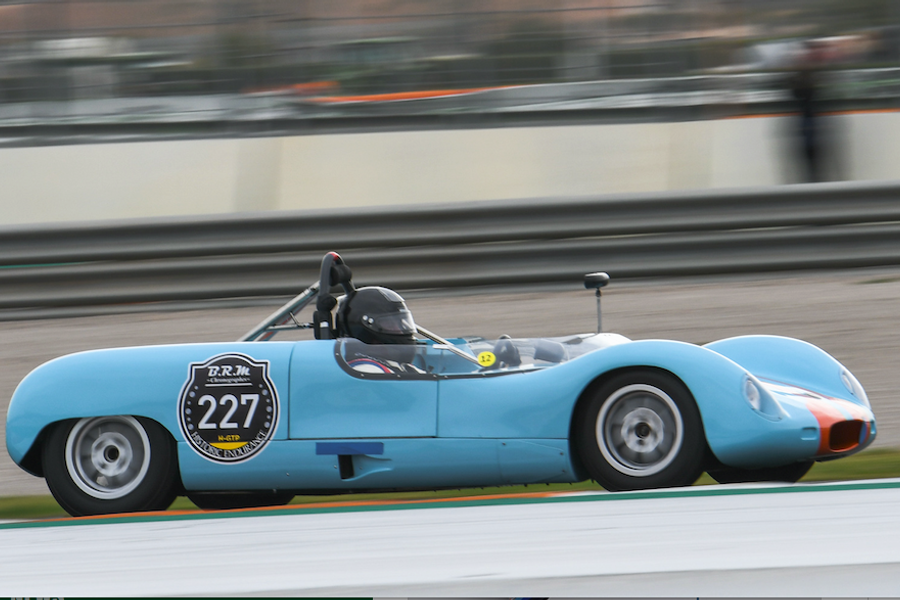This dynamic, angled close-up captures a bright blue convertible race car speeding along a racetrack. The car, which has a sleek and sloped front end featuring a red stripe at the tip of the nose and a black grille, is adorned with a round black sticker towards the back quarter panel with the number 227 in white and some unreadable text. The image focuses on the driver, who is wearing a black helmet with a clear visor and a white shirt secured by red seatbelts. The helmet obscures the driver's face. The car's black wheels with silver interiors are also blurred, enhancing the sense of high velocity. In the foreground, the gray racetrack is visible with a green stripe along one side, while the background remains a blur, emphasizing the car's rapid movement.